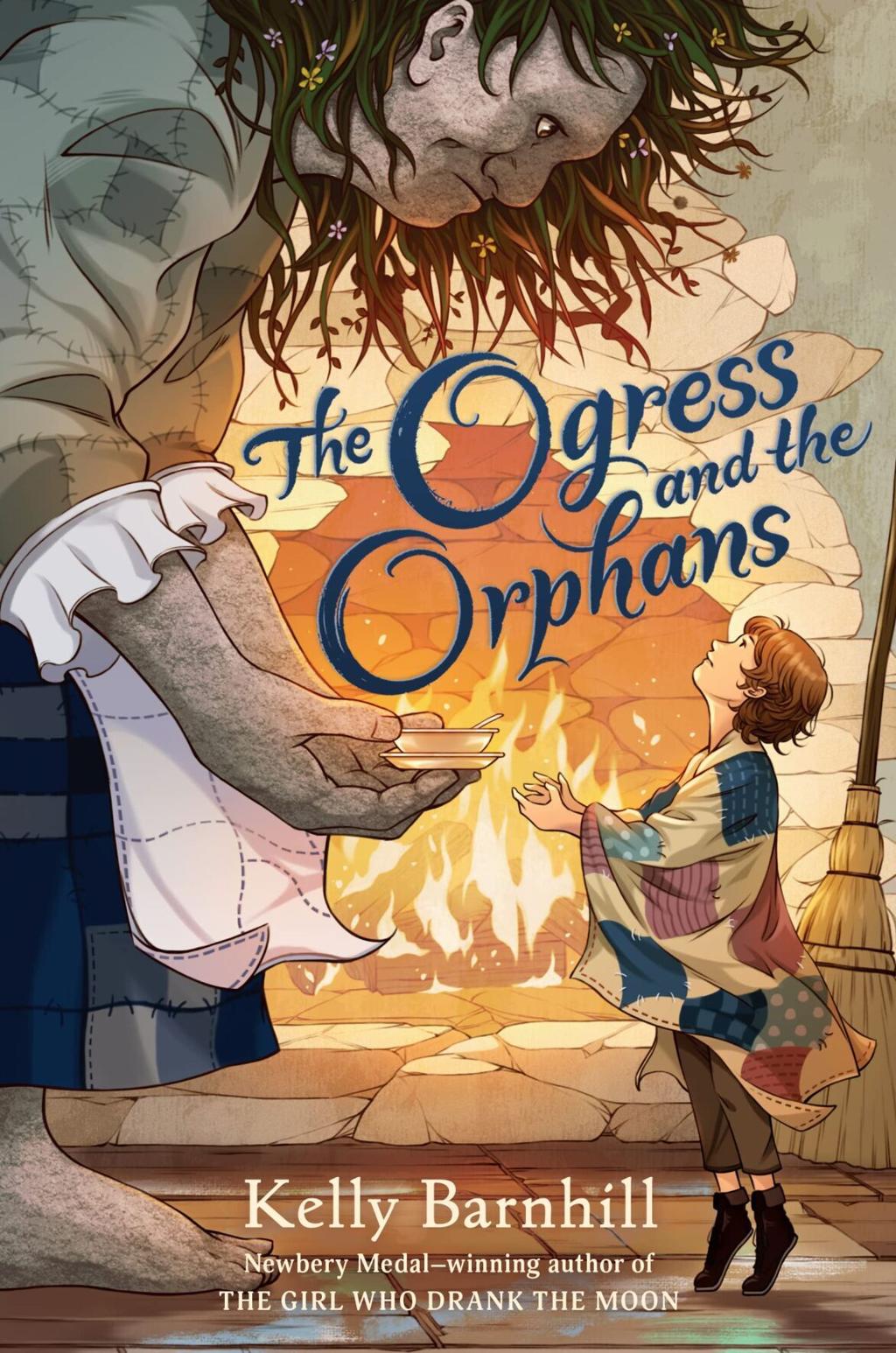This is a detailed illustration of the book cover for "The Ogress and the Orphans" by Kelly Barnhill, the Newbery Medal-winning author of "The Girl Who Drank the Moon." The scene prominently features a towering, pale-skinned ogress on the left, dressed in a blue-gray checkered skirt and a grayish-white top, over which she wears a white apron. Her long dark hair is adorned with yellow and purple flowers. She is bending down with a warm, friendly smile, offering a steaming bowl of soup to a young boy. The boy, wrapped in a tattered blanket or quilt over short brown pants, stands on his tiptoes and looks up at her. Notably, he wears only socks—no shoes. The setting around them includes a large broom that almost matches the boy in size and a roaring brick fireplace that adds warmth to the scene. The hearth and brick floor underfoot complete the cozy ambiance. The title, "The Ogress and the Orphans," is displayed prominently in blue text above the heartwarming interaction, with “Kelly Barnhill, Newbery Medal-winning author of The Girl Who Drank the Moon” noted at the bottom.